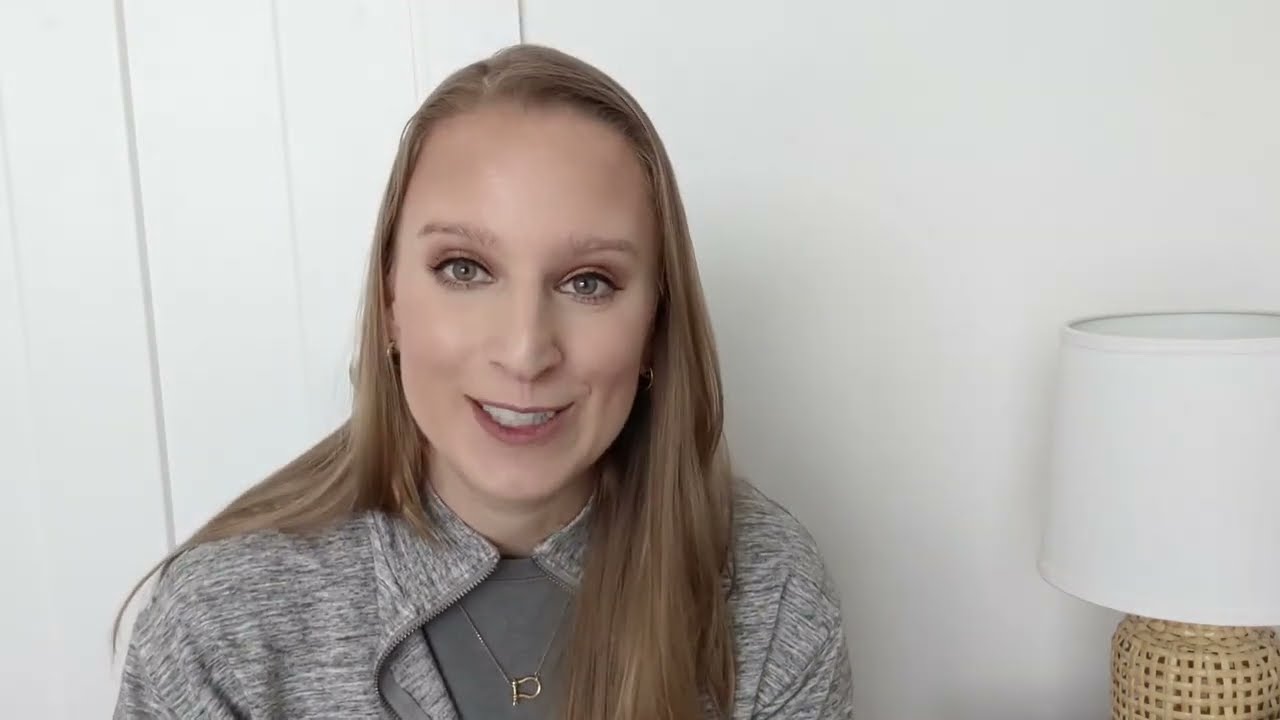The photograph features a woman centered in the frame at chest to shoulder level. She has long, light brown, almost blonde hair that cascades both in front and behind her shoulders. Her hazel eyes, which may appear slightly grayish-blue in certain lights, stand out along with her prominent nose and cheekbones. She is wearing a light grey overcoat or zip-up sweater over a grey t-shirt. Her ensemble includes small gold hoop earrings and a distinctive necklace with a pendant resembling a golden pea. The woman, who is either smiling or in mid-speech, exposes both her top and bottom teeth. Her expression suggests she might be interacting with the camera as part of a video. The background is primarily a white wall, and to her right, there is a table lamp with a wicker-patterned light brown base and a white lampshade. To the left, the background appears to include white paneling or possibly blinds, contributing to the clean, minimalistic setting.